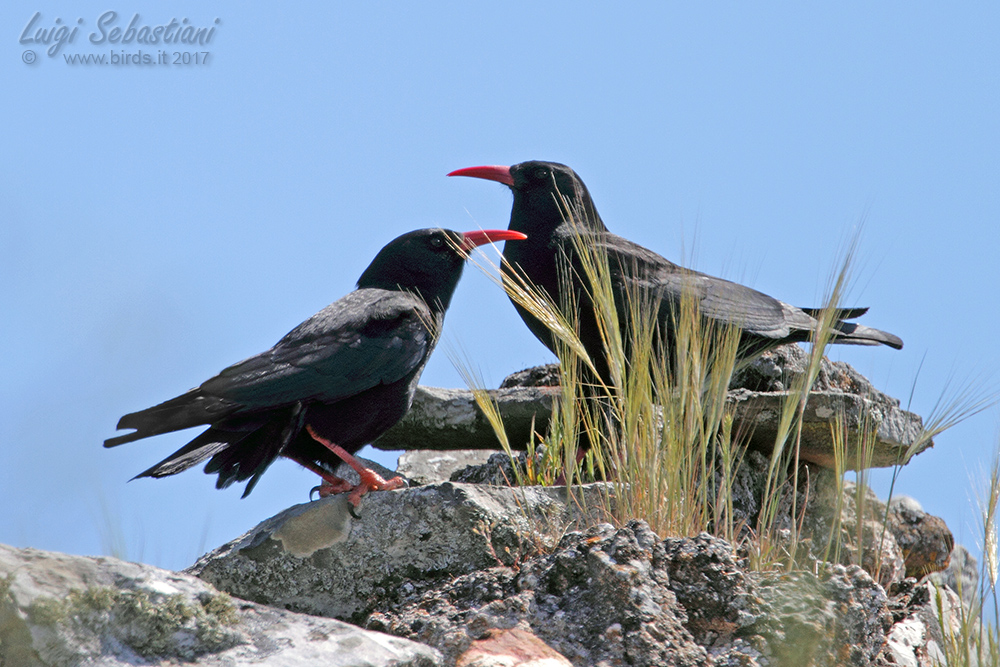This photo captures a serene moment in nature with two birds perched on rocks amidst a clear blue sky backdrop. The larger bird in the background and the slightly smaller one in the foreground are both primarily black with touches of white on their feathers. Each bird has distinctive orange legs and feet, and vivid reddish-orange beaks. The birds are positioned on different rocks, with the larger bird facing left and the smaller bird facing right, perhaps suggesting an interaction or a watchful gaze over its young. 

The rocks are piled up, seemingly on a high point such as a hillside or cliffside. Tufts of grass jut out from between the rocks, adding a touch of green to the scene. The setting is clearly outdoors in daylight, captured brilliantly against the vivid blue sky. 

In the top left corner of the image, faint black text reads 'Luigi Sebastiani' and 'www.birds.it 2017,' providing credit and context for the photo. The harmonious blend of colors—blue, black, red, gray, and hints of orange—along with the natural setting, makes this an engaging picture for bird lovers and nature enthusiasts alike.